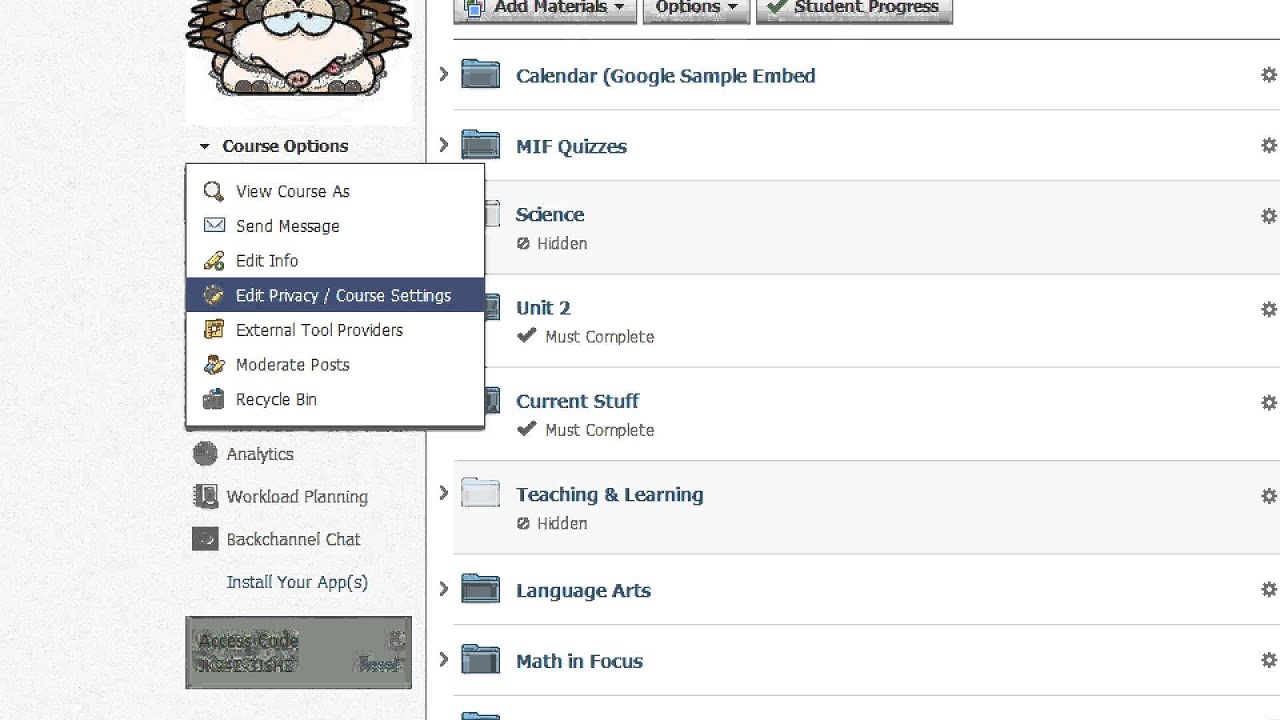The image depicts a vintage website interface reminiscent of mid-1990s web design, characterized by its blocky layout and simple graphics. The website is slightly wider than it is tall, with the left third of the screen dedicated to navigation on a gray background. 

At the top left, there is a cartoon animal avatar with a pink nose and brown spikes protruding from both sides of its head, facing forward. Below this cartoon figure, the navigation menu lists various options. The section titled "Course Options" is expanded, revealing a drop-down box with a white background and multiple selection items.

The drop-down includes:
- "View Course"
- "Send Message"
- "Edit Info"
- "Edit Privacy / Course Settings" (highlighted with a blue background indicating it is currently selected)
- "External Tool Providers"
- "Moderate Posts"
- "Recycle Bin"
Unselected items further down the list are:
- "Analytics"
- "Workload Planning"
- "Back Channel Data"
- "Install Your Apps (S)"

On the right side of the screen, additional selectable elements are visible, including links to "Quizzes" and a "Calendar." The overall aesthetic is minimalistic and functional, a clear nod to early internet designs.